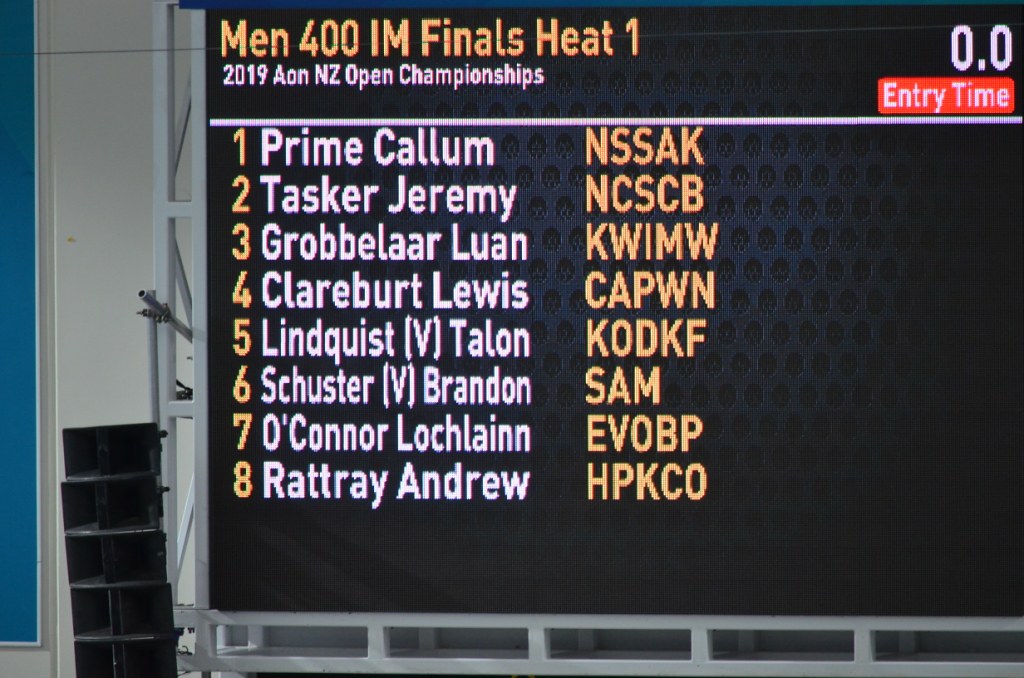This image prominently features a black scoreboard capturing the details of the men's 400 IM finals, Heat One, at the 2019 AONNZ Open Championships. The scoreboard covers most of the frame, with a thin slice of a white wall and a blue vertical stripe visible along the left edge. The scoreboard text includes "Men 400 IM Finals Heat One" in striking orange letters, and "2019 AONNZ Open Championships" in white below it. In the upper right corner, a white "0.0" is displayed. A red rectangle with white text marked "Entry Time" is positioned below. Beneath this are the names of the competitors, with positions in yellow and names in white. The entries read: 
1. Prime Callum (NSSAK),
2. Tasker Jeremy (NCSCB),
3. Groblar Loon (KWIMW),
4. Clarebert Lewis (KAPWN),
5. Lindquist, V. Tallon (KODKF),
6. Schuster, V. Brandon (SAM),
7. O'Connor, Loughlane (EVOBP),
8. Ratray Andrew (HPKCO).